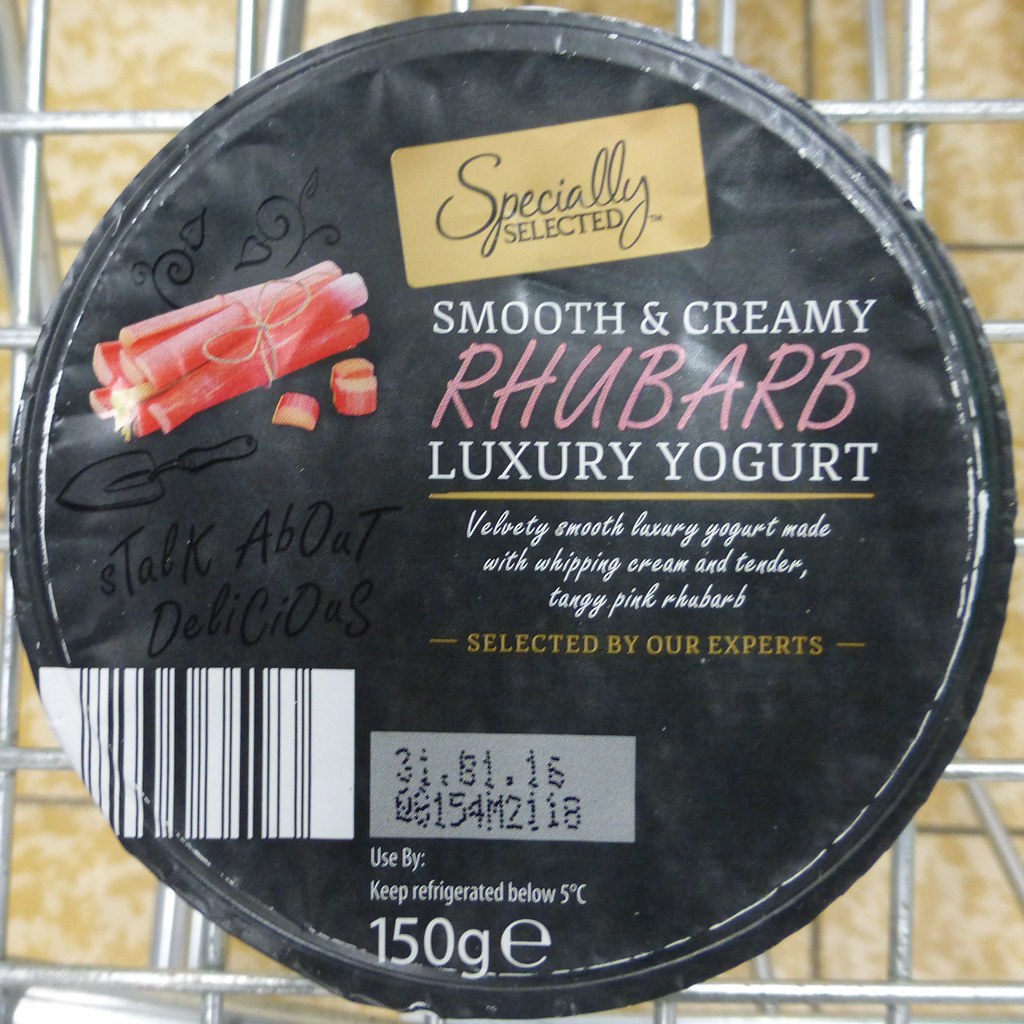The image displays the top of a circular yogurt container with a peel-off lid. The lid is black and prominently features the text "Specially Selected Smooth and Creamy Rhubarb Luxury Yogurt." Detailed descriptions include "Velvety smooth luxury yogurt made with whipping cream and tender tangy pink rhubarb selected by our experts." A playful font on the side reads "Talk about delicious." Adjacent to the text, there is an artistic illustration of red rhubarb stalks tied together with twine, accompanied by some sliced rhubarb and tendrils, along with a gardening trowel. Additional text includes a "use by" date marked as "31.01.16" and storage instructions stating "keep refrigerated below 5 degrees Celsius." The container also weighs 150 grams. The yogurt lid appears to be resting on metal grates, possibly within a shopping cart or basket.